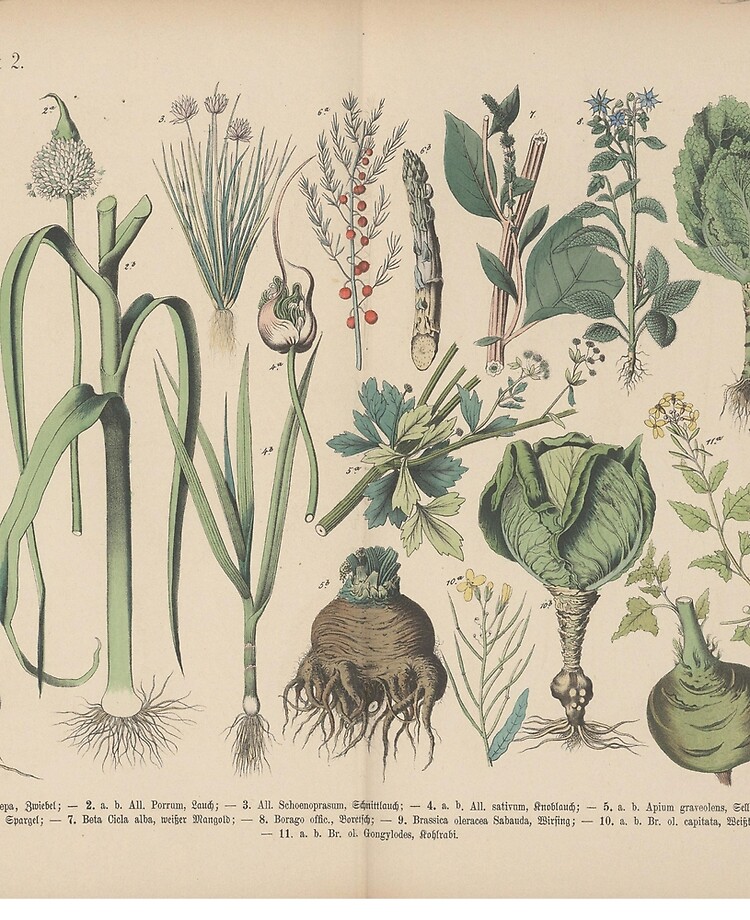This image depicts a page from what appears to be an old, possibly German, textbook on plants, showing detailed illustrations of various plant types. The page features eleven meticulously sketched plants, mostly in shades of green, with visible roots, stems, leaves, and occasional flowers. Each plant illustration is accompanied by a number that correlates to detailed descriptions found at the bottom of the page. The text, written in small print and not in English, possibly German, includes names and classifications for each plant. The descriptions at the bottom are formatted with numbers and include specific plant names such as asparagus, turnips, onions, celery, and other vegetables or weeds. The page shows signs of wear, with a prominent fold in the center, suggesting it might have been taken from a dated textbook. This layout functions similarly to a chart, where each numbered plant matches an explanatory passage, much like a labeled key. The illustrations display diverse plant features, including white flowers, leafy greens, and bulbous roots, highlighting both common vegetables and possibly some lesser-known species.